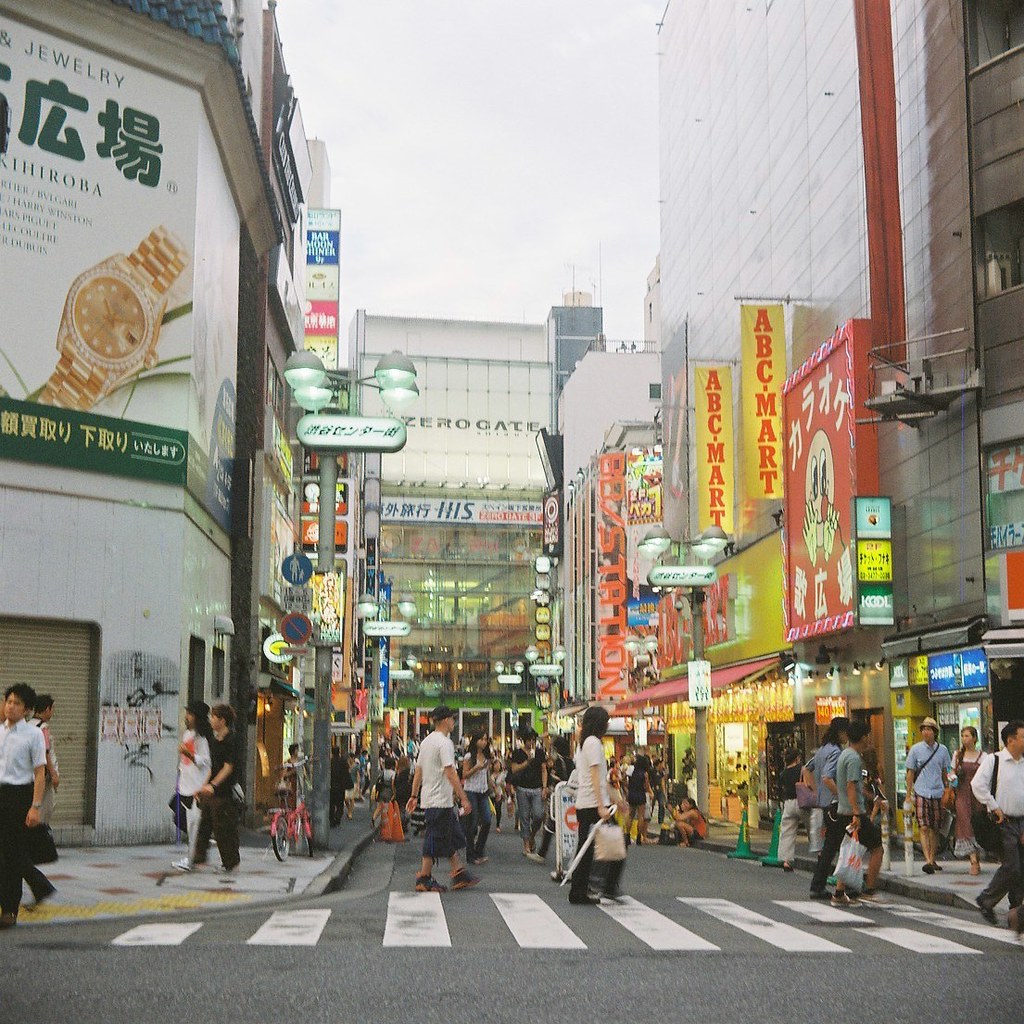This highly detailed photograph captures a bustling intersection in what appears to be an older, slightly worn yet vibrant Japanese city. The streets are teeming with people, predominantly of Asian descent, moving in all directions—many in the crosswalk and others along the sidewalks. The weather is sunny and clear, though a few individuals carry umbrellas along with shopping bags and groceries, adding to the lively atmosphere. The scene is dominated by numerous storefronts and buildings adorned with a plethora of signs, lit up with neon lights and light bulbs—in an assortment of colors, creating an overwhelming yet beautiful visual tapestry. Prominent among these signs is a large billboard on the left featuring a gold watch, alongside a more understated sign for ABC Mart on the right. The entire street emits a sense of organized chaos, filled with younger individuals, single pedestrians, and couples, all contributing to the dynamic and spirited scene of this Japanese city street.